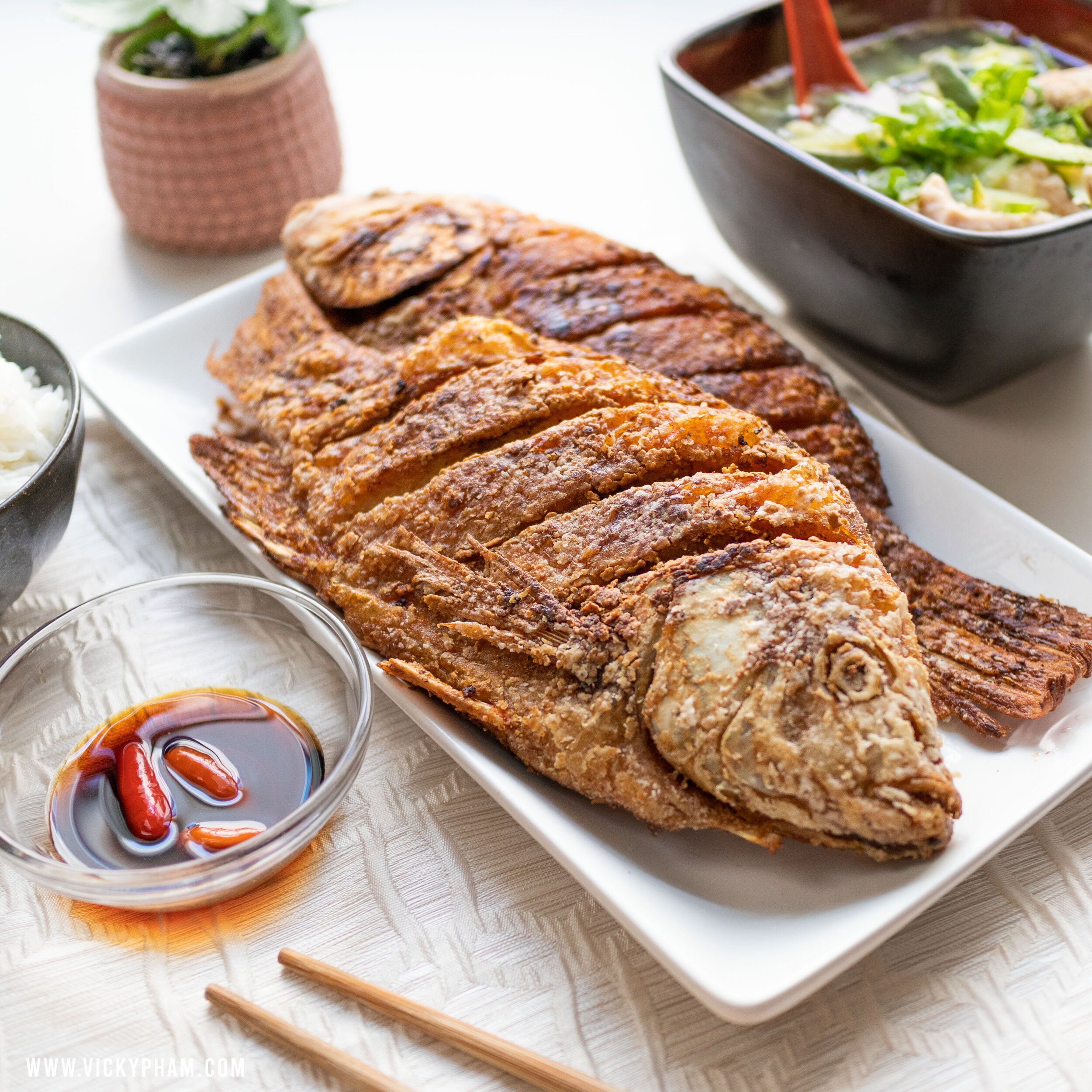The photograph captures a well-presented meal featuring two fully intact, crispy, fried fish served on a white rectangular plate. The fish are arranged with their heads and tails alternating, showcasing their brown, seasoned exterior. Surrounding the main dish are several other items: to the right of the fish lies a square-shaped bowl of soup containing visible green onion and various vegetables, with possible pieces of chicken. To the left, a small bowl of sauce, which appears to be a soy-based mixture with chili, provides a flavorful accompaniment. Just barely visible at the top left edge of the image is a white bowl of rice. The table, adorned with a patterned tablecloth, also features partially shown chopsticks at the bottom of the photo. The background of the tablecloth fades into a nearly white color, giving emphasis to the vibrant and detailed meal.